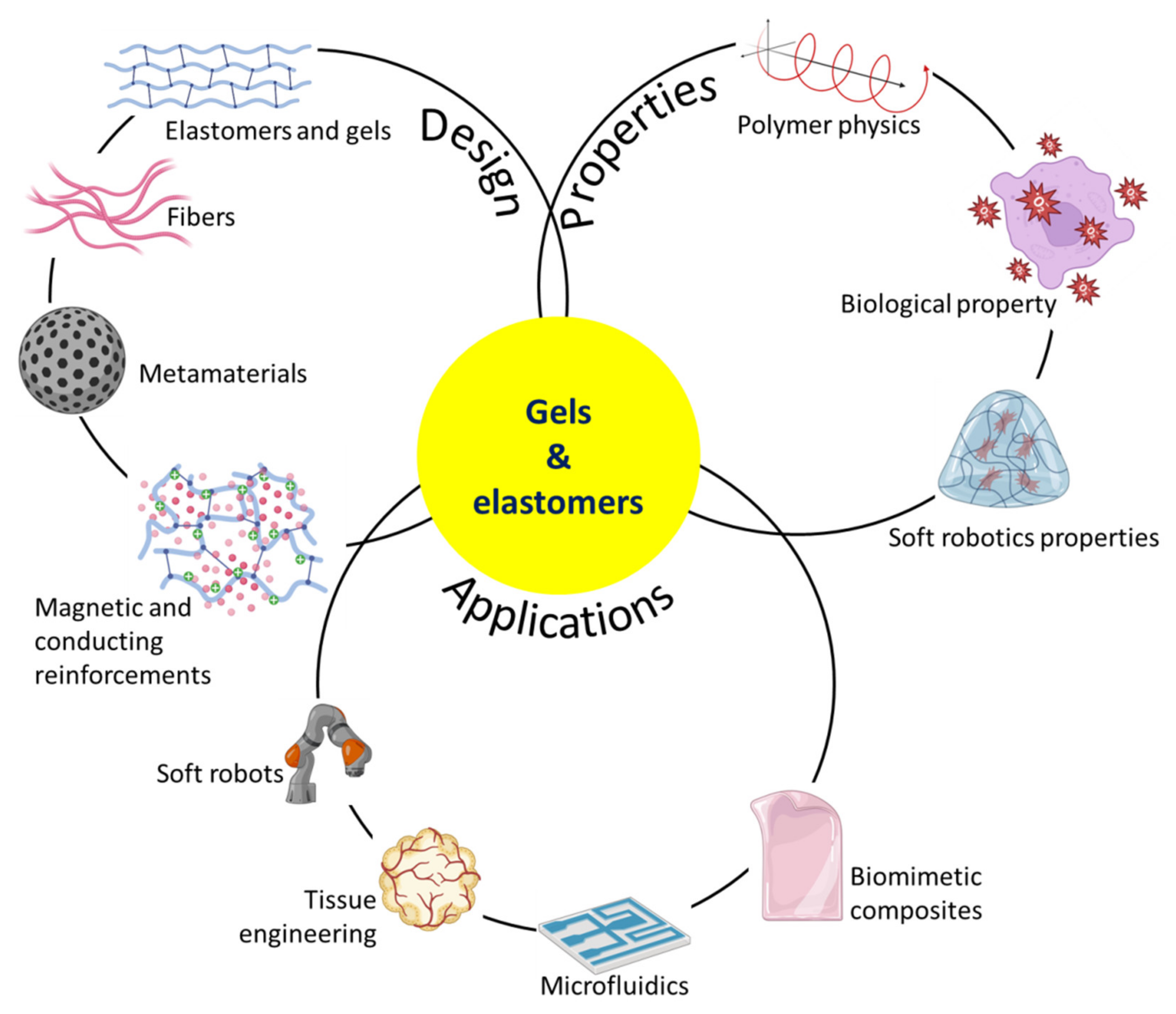This is a detailed Venn diagram with three main circles labeled: Design, Properties, and Applications, set up in a triangular arrangement with two circles on top and one on the bottom. In the center, overlapping all three circles, is a prominent yellow circle labeled "Gels and Elastomers." 

The Design circle contains elements such as elastomers and gels, fibers, metamaterials, and magnetic and conducting reinforcements. The Properties circle highlights polymer physics, biological properties, and soft robotics properties, each accompanied by a representative symbol. The Applications circle features soft robots, tissue engineering, microfluidics, and biomimetic composites, also illustrated with individual icons.

Overall, the diagram interconnects these categories, emphasizing how "Gels and Elastomers" are central to the design, properties, and application aspects, making it a comprehensive visual from a scientific context likely found in a textbook.